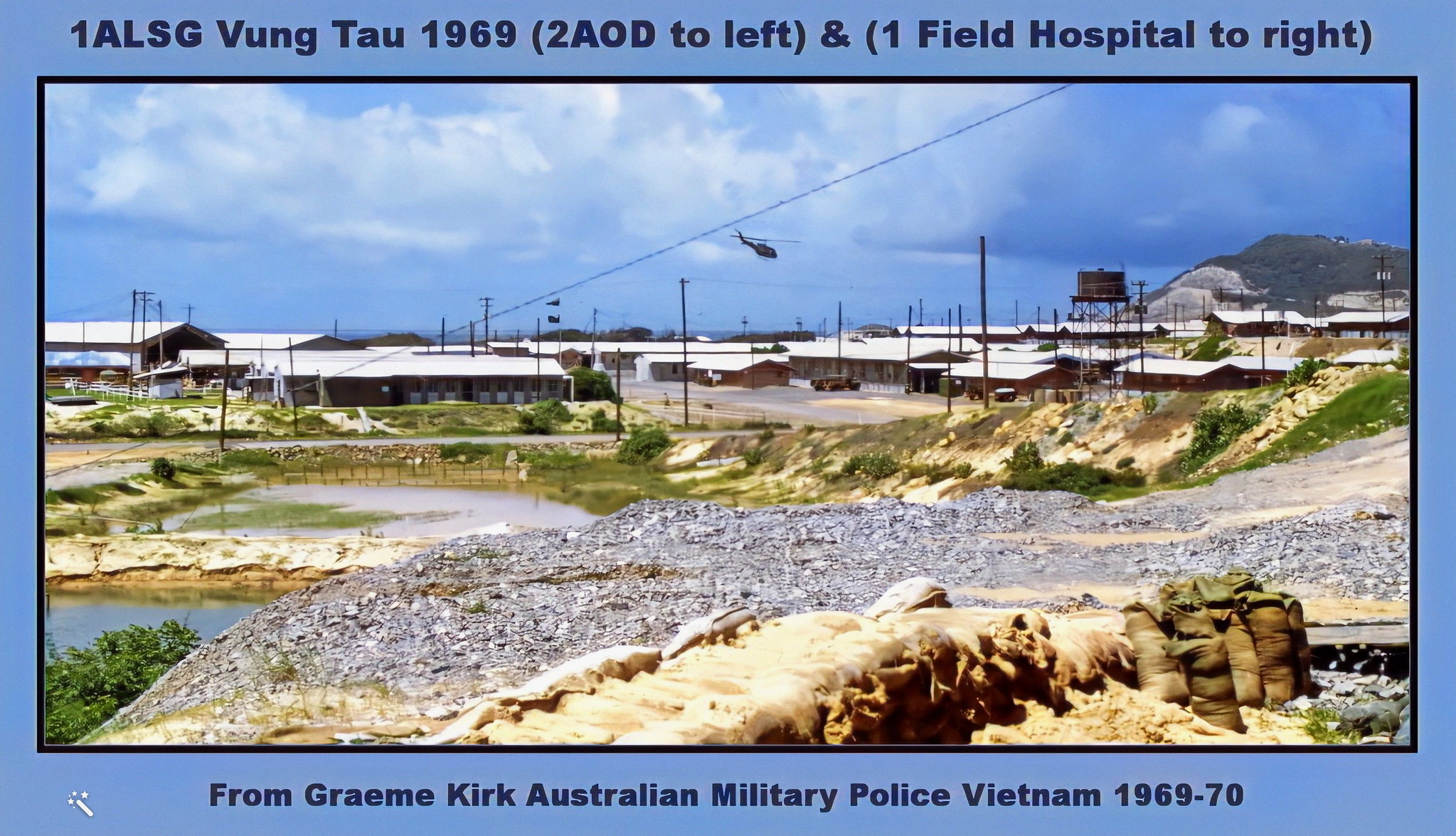This postcard-style photograph is set against a dark blue border and framed by a thin black outline. At the top of the border, in neatly printed black text, it reads "1 ALSG Vung Tau 1969 (2 AOD to left) (1 Field Hospital to right)". The border's footer states, "From Graham Kirk, Australian Military Police, Vietnam 1969-70," and features a white magician's wand with three stars in the lower left-hand corner.

Inside the black border lies the main photograph, rectangular and landscape-oriented. The scene captures a military camp, presumably in Vietnam, suggested by the captions. Dominating the foreground is a mound of sandbags extending from the center bottom to the right-hand corner, leading up to a gravelly, slightly raised road. Scattered water pits and a muddied grassy area become visible as the terrain extends back.

The background reveals several military buildings, mentioned in the text, with a telephone pole, power lines, and a water tower on the right-hand side. Hovering in the top portion of the image is a helicopter, seemingly suspended in mid-air against a backdrop of a blue sky dotted with large whitish-blue clouds, which darken towards the right. The scene subtly conveys a slice of everyday life at a military post during the Vietnam War.